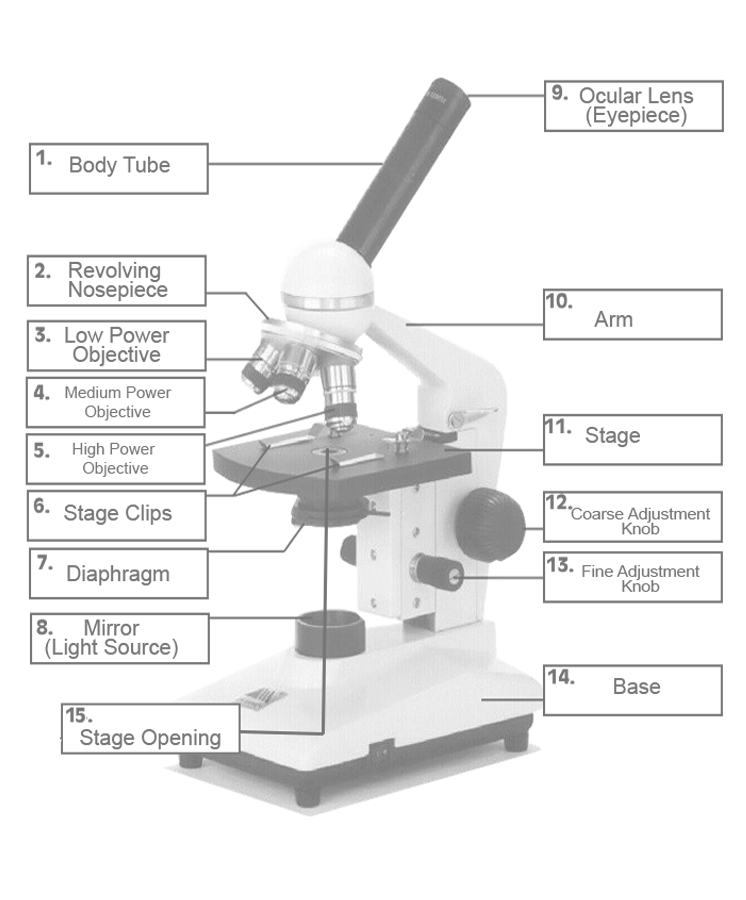The image is a detailed black and white photograph of a single eyepiece, compound microscope, presented at a slight leftward angle. The microscope features three revolving lenses (low, medium, and high power objectives) mounted on a revolving nose piece. The eyepiece is directed towards the top right of the image. The parts are meticulously labeled with numbered black-bordered rectangles, accompanied by black text. The descriptive text runs from 1 to 15, with labels positioned on both sides of the microscope. Key components include the body tube, stage clips, diaphragm, mirror light source, and stage opening—all contributing to its functionality. The microscope, primarily white with black trimmings, stands on rubber feet for stability. Notable features include the course and fine adjustment knobs for focusing, and a robust base, ensuring firm support. The detailed labeling showcases the body tube (1), revolving nose piece (2), low (3), medium (4), and high power objectives (5), stage clips (6), diaphragm (7), mirror/light source (8), ocular lens eyepiece (9), arm (10), stage (11), coarse adjustment knob (12), fine adjustment knob (13), base (14), and stage opening (15).